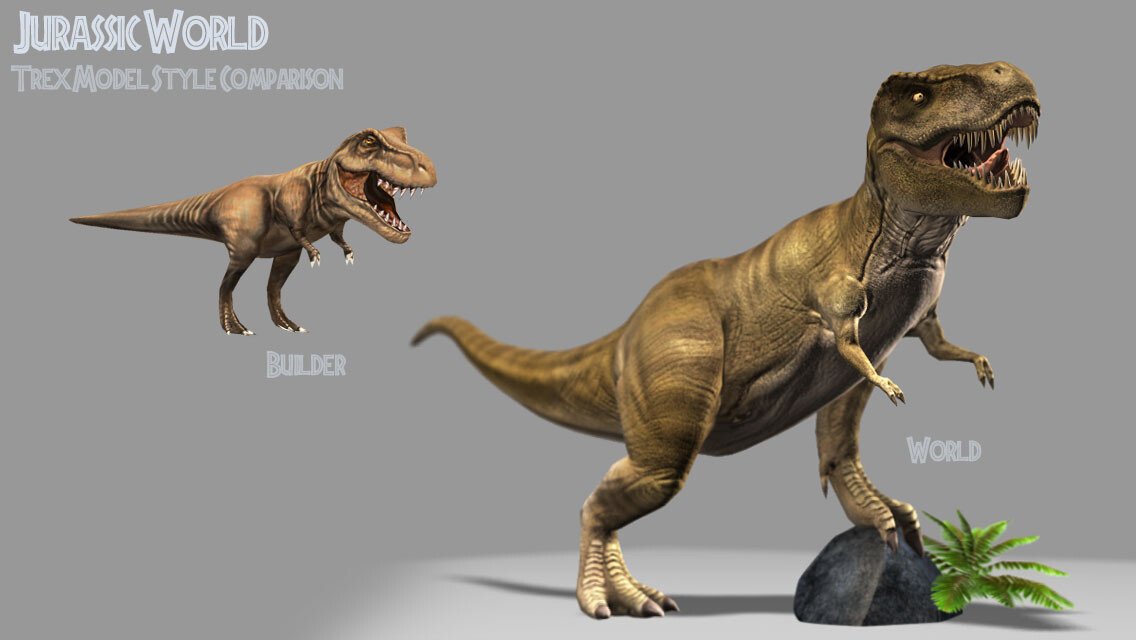This CGI image presents two T-Rex models against a predominantly medium grey background, with a slightly lighter grey illumination in the bottom right corner. Positioned prominently on the right side is a detailed T-Rex model with greenish-brown rough skin, large head, open mouth showcasing sharp teeth and a pink tongue. It has distinct yellow eyes with striped black and green ridges above them, and stubby pale yellow arms each ending in two black pointed tips. This T-Rex stands with its left leg on a grey rock, accompanied by a green fern beside it, while its right leg is grounded. Its long, pointed tail extends into the distance, slightly blurred.

On the top left corner is a smaller T-Rex model of similar appearance but with a more reddish-brown skin tone. Above this smaller dinosaur, the text reads, "Jurassic World T-Rex Model Style Comparison," with the titles "Builder" beneath the smaller dinosaur and "World" beneath the larger, more detailed one. The meticulous detailing on the larger model suggests it represents the final T-Rex design used in the "Jurassic World" film, whereas the smaller model appears to be an initial concept or preliminary version.